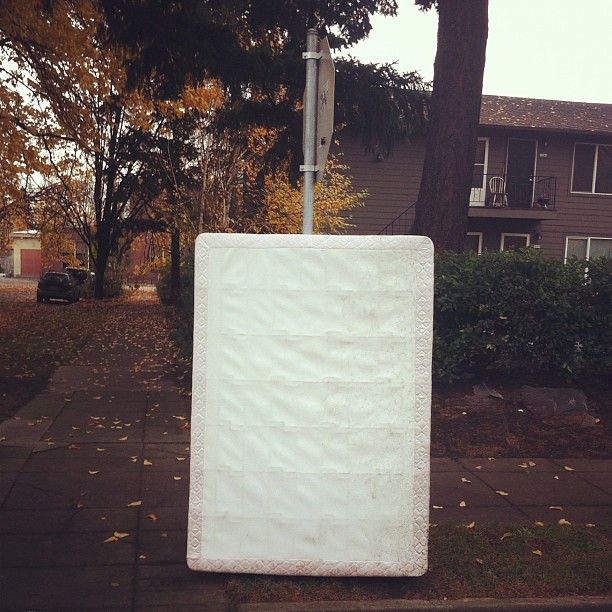The image depicts an autumn street scene viewed from the side of a building, with leafy trees shedding orange and yellow leaves onto the sidewalk. On the left, several cars are parked along the street. Dominating the center right of the image is a tall, dark brown tree trunk. Behind this tree stands a two-story, dark brown house with a red, sloping roof speckled with fallen leaves. The house features a small balcony with wire railings, a white chair, and an aluminum door. Bushes line the front of the house. A large white mattress leans against a stop sign, its pole barely visible against the backdrop of the hedge and the house. The scene is dotted with various street elements like garages and additional buildings, creating a quintessential urban autumn landscape.